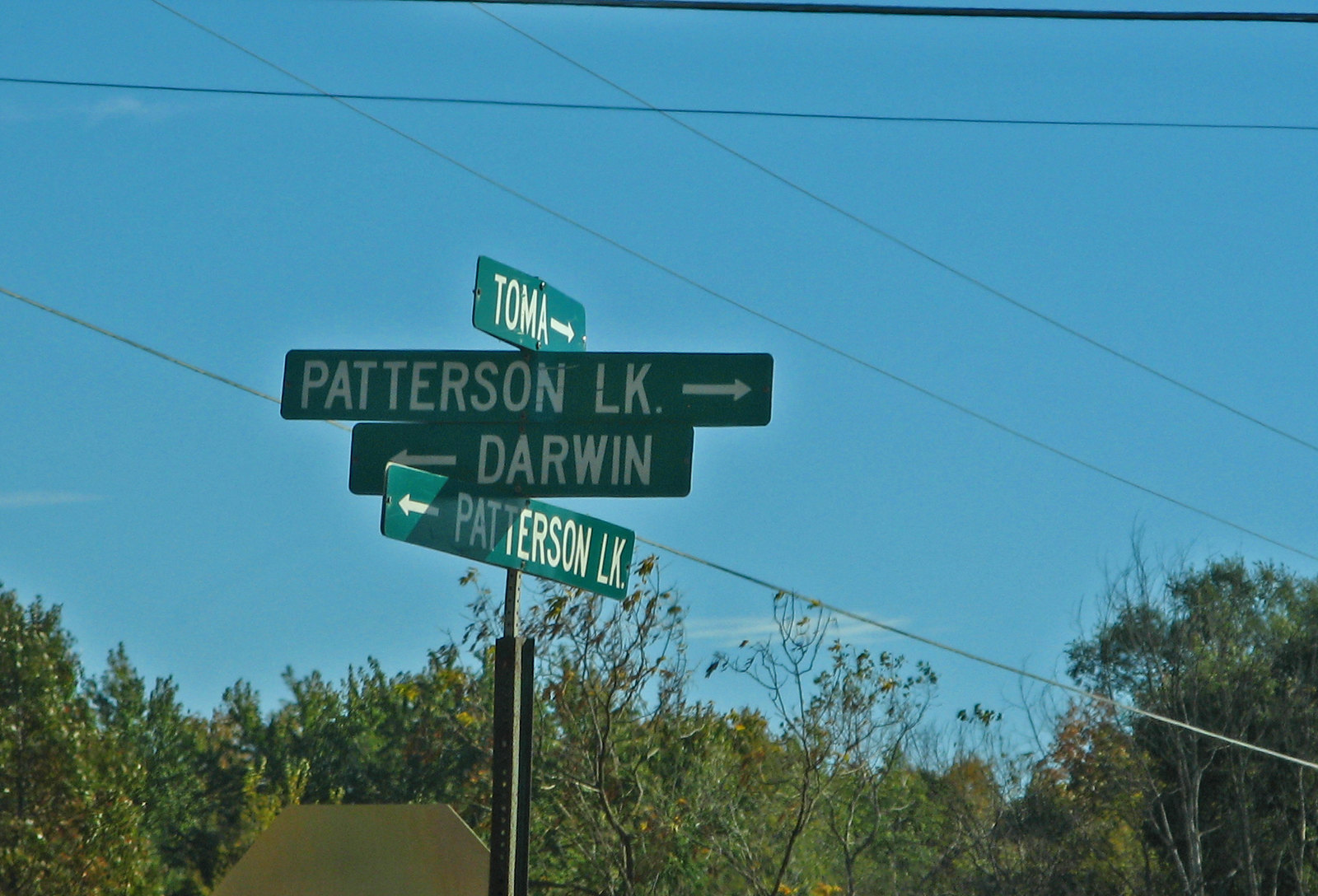The image captures a clear, sunny day at what appears to be a suburban or rural street intersection. The sky is bright blue with few clouds. Power lines crisscross overhead, and the tops of multiple trees—some green and leafy, some dormant—are visible. A stop sign can be seen from behind, and there is a prominent street sign post displaying four street names. The names are Tomah, Patterson Lake (repeated two times in different directions, indicating it spans both ways), and Darwin. This intersection is marked with Tomah pointing forward, Patterson Lake pointing right and backward, and Darwin pointing left. The scene lacks buildings, emphasizing the tranquility and openness of the setting.